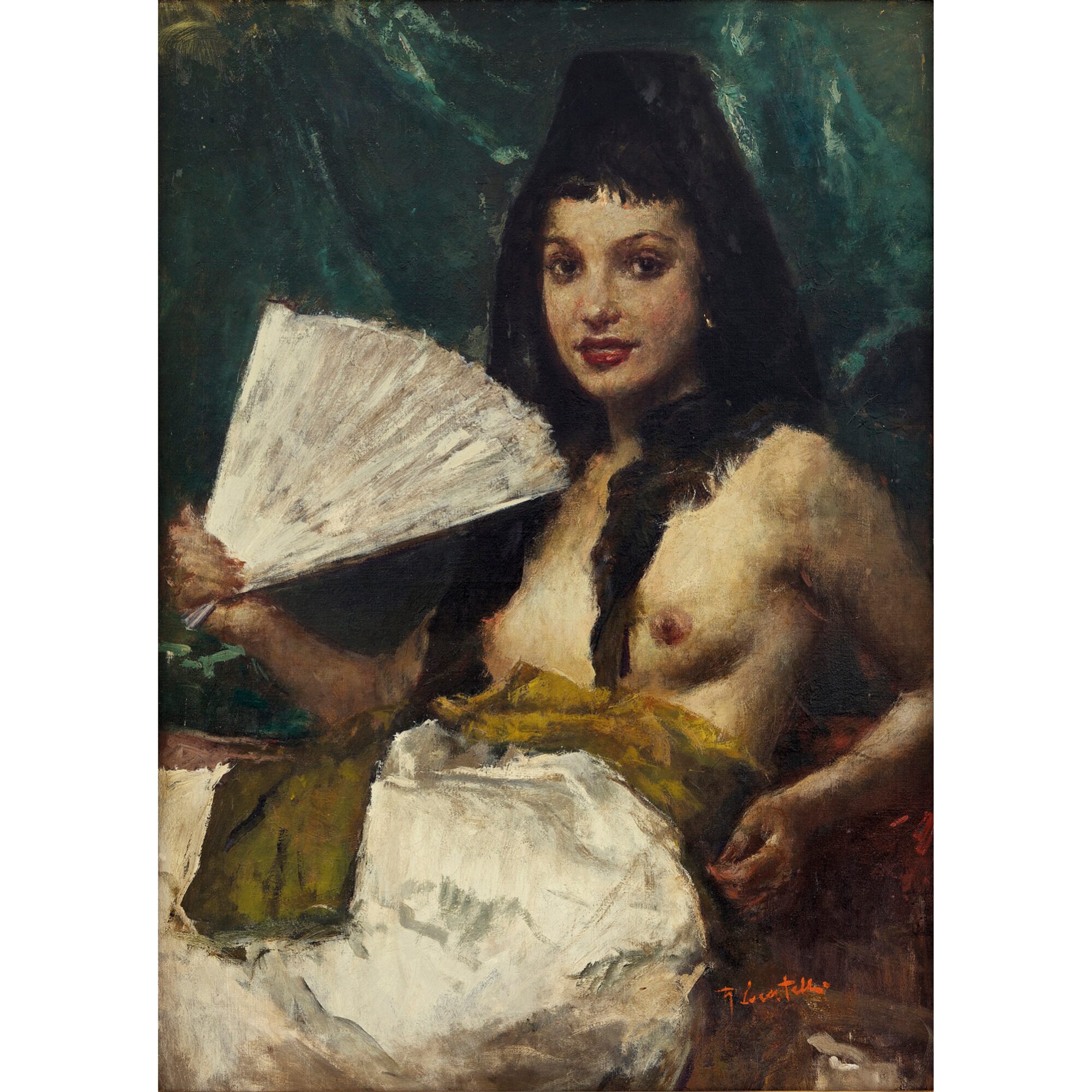The painting, likely an abstract watercolor or oil piece, portrays a semi-reclining woman who appears to evoke the likeness of Cleopatra. Bare from the waist up, she is draped in a white and yellow robe or skirt from the waist down. Positioned slightly to the right of the center, she gazes with a subtle smile, her dark eyes and very long black hair—swept over both shoulders—creating an alluring visage. Her lips are vividly red, contrasting with her light skin. In her left hand, she holds a partially unfurled white fan pointed towards herself. She reclines on a dark brown cushion or chair, with an abstract background of dark and light teal, dark green, blue, and hints of gold at the top left corner. The bottom right of the image features the artist's signature in bright orange, adding a striking detail to the composition.